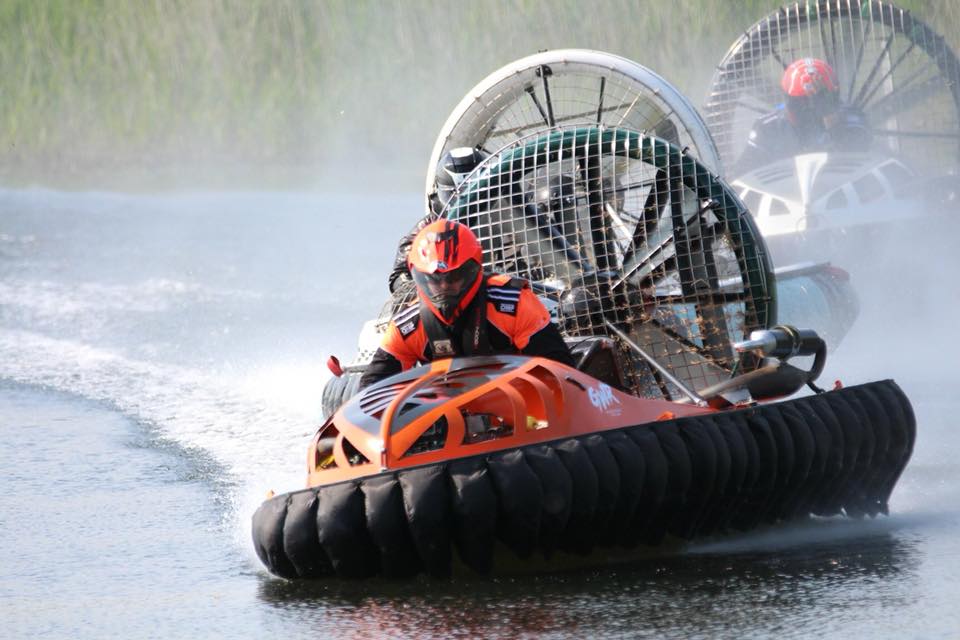In this dynamic outdoor image, three racers are participating in a hovercraft race over a large, slightly wavy body of water, possibly a lake or river, surrounded by tall grass and distant forests. The lead racer is prominently visible, wearing an orange helmet and an orange and black jumpsuit with white stripes. His hovercraft features a matching orange and black color scheme, with a black and green fan propelling it from the back. Trailing behind him are two more racers, partially obscured by water spray and mist. 

The second racer is less visible, hidden behind his hovercraft's white fan, while the third racer's details are clearer: he wears a red helmet and a black jacket, operating a white and black hovercraft with a black and blue fan. All three racers are captured mid-turn, emphasizing the action and speed of the competition, with water misting around them, adding to the sense of motion and excitement.